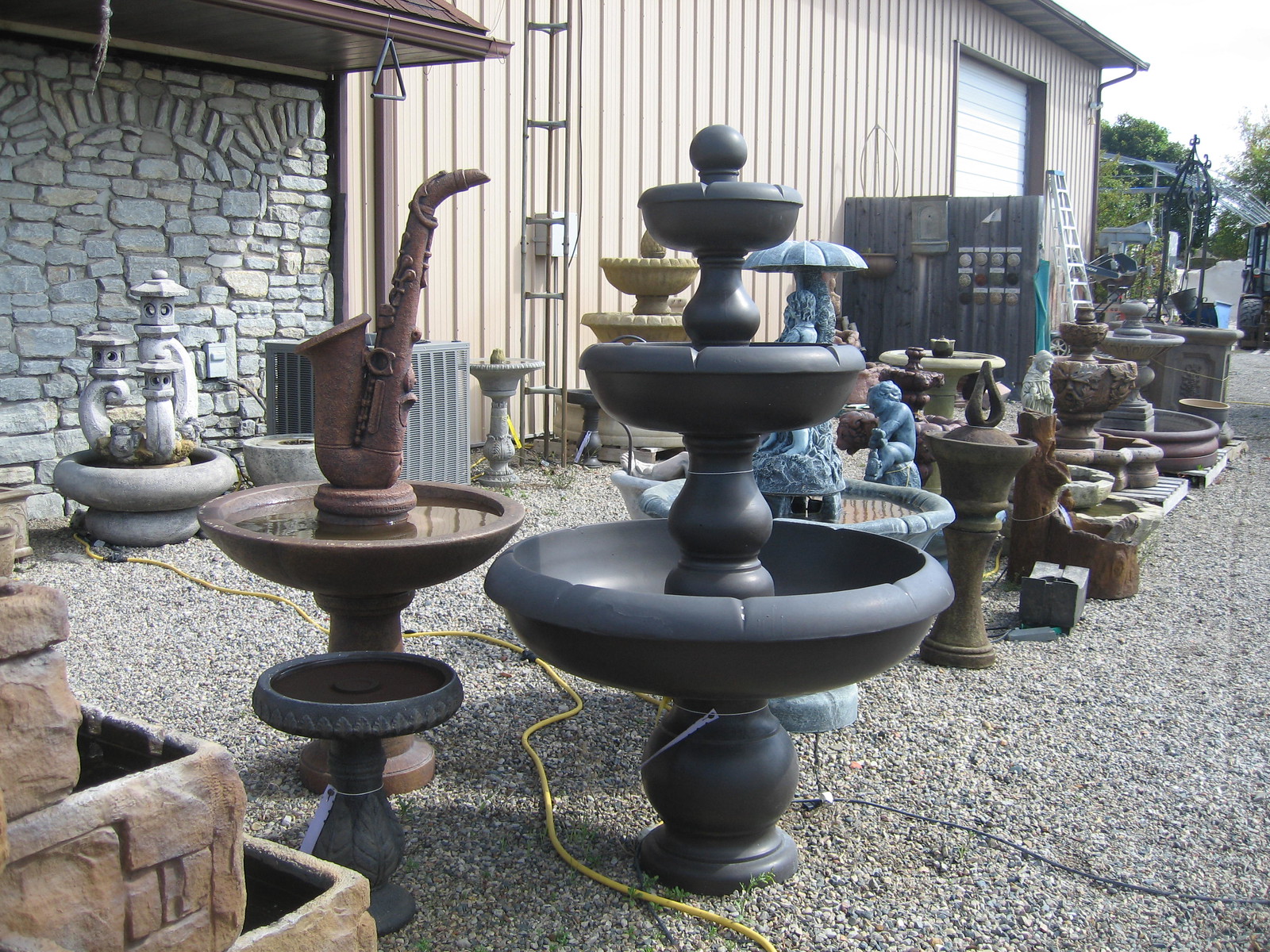The image captures a vibrant outdoor display of garden fountains and birdbaths located at a garden center or concrete shop. These unique fountains, each distinctly different, are positioned on gravel pathways outside a large building. The largest gray fountain features a chalice-upon-chalice design with a decorative knob at the top. Among the other noteworthy pieces, there is a birdbath with a saxophone centerpiece, a three-layer black fountain, a sculpture of a couple beneath an umbrella, and an Asian-inspired fountain in the shape of pagoda-like toadstools.

The setting includes a warehouse with tan vertical metal siding, a tall white overhead garage door to the right, and a stone wall with archways to the left. The gravel yard is dotted with extension cords and pallets, and a ladder leans against the building near the garage door. Visible in the background are the metal structures of a greenhouse and a tall radio antenna, hinting at the expansive nature of the premises. The foreground features additional garden equipment, including a heat pump unit and various garden sculptures, all contributing to the bustling atmosphere of the sales yard.